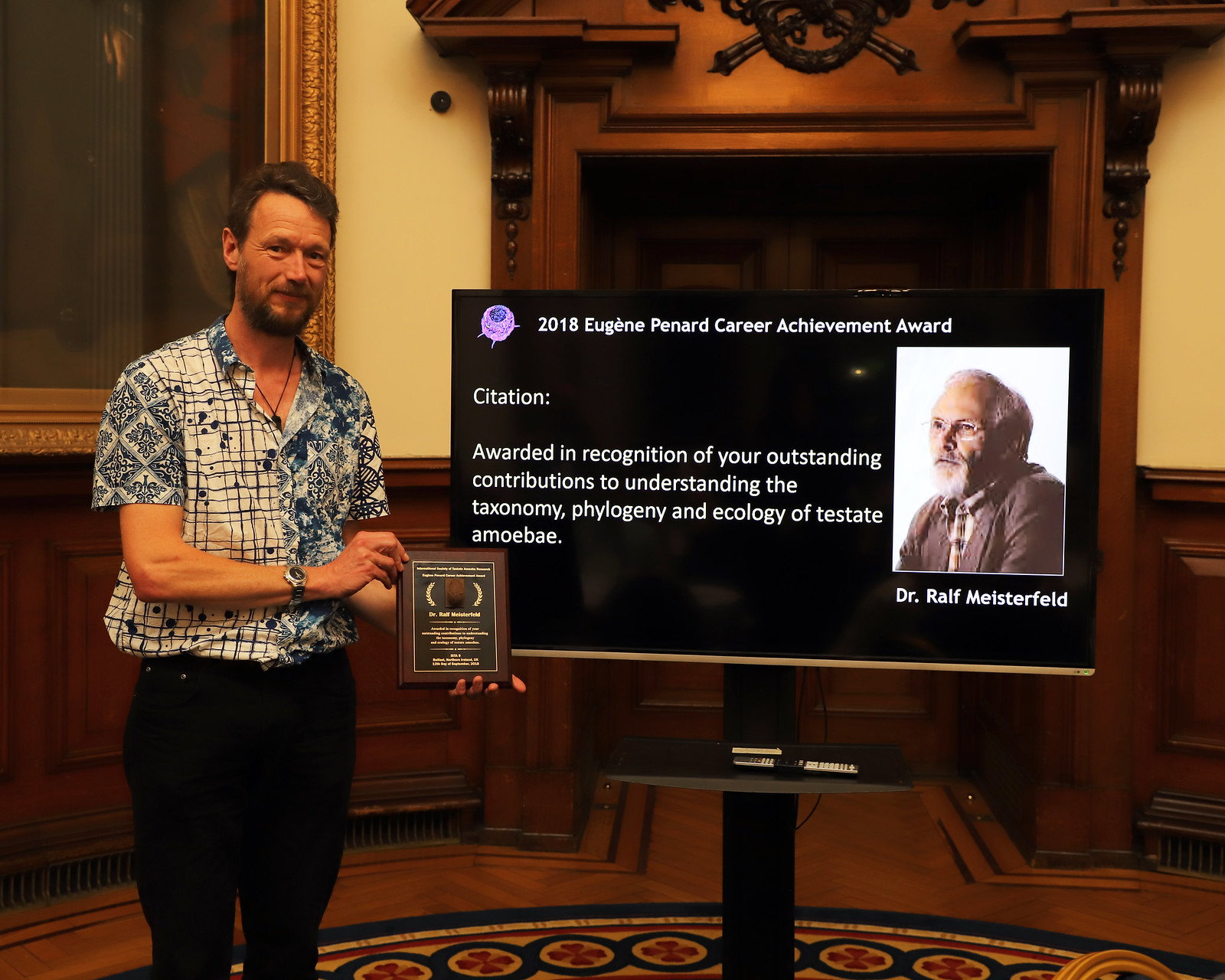In the photograph, a bearded man with a joyous expression is holding a wooden plaque and posing in front of a large television screen. The screen displays white text which reads, "2018 Eugene Prenard Career Achievement Award," followed by, "Citation: awarded in recognition of your outstanding contributions to understanding the taxonomy, phylogeny, and ecology of testate amoebae." The man, identified from the partially readable plaque as Dr. Ralph Maysterfield, is visible from his knees upwards. He is dressed casually in tight black jeans and a loose-fitting blue button-up shirt with the top two buttons undone. He also wears a necklace and a silver watch. The interior setting is an elegant, old-fashioned room with a rotunda-like ambiance. It features a wooden floor with a round rug, wood paneling, and an ornate, vintage painting on a yellow wall to the left. A large wooden-framed doorway can be seen, adding to the classic aesthetic of the space. Additionally, there is a photograph of a bald man wearing glasses, identified as Dr. Ralph Meisterfeld, displayed on the television screen.